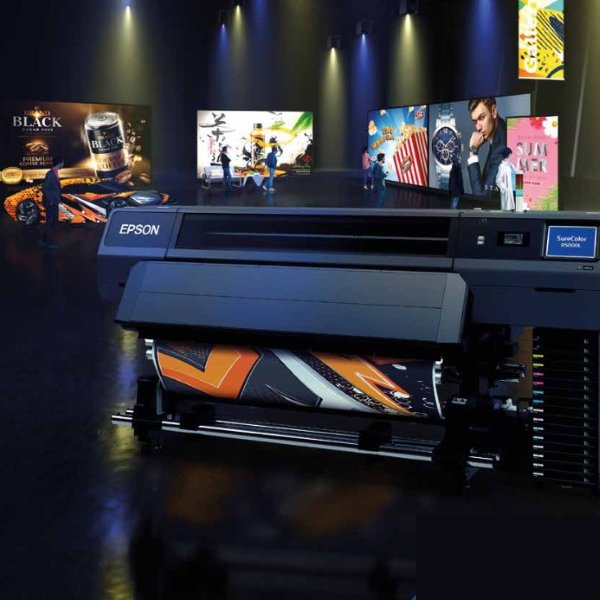The image features a black Epson printer prominently in the foreground, situated on a black, slightly reflective surface. The printer is in the process of printing a dark-colored photo. Notably, the printer displays the Epson logo in the upper left corner and a blue label on the right side. In the background, the setting appears to be a gallery or museum, illuminated by alternating yellow and blue spotlights shining down on various images. These images include an advertisement featuring a beer can labeled "black", a photograph of a man in a black suit, and another of popcorn against a pink background among others. The surrounding area shows people walking through the gallery, viewing the displayed photographs.